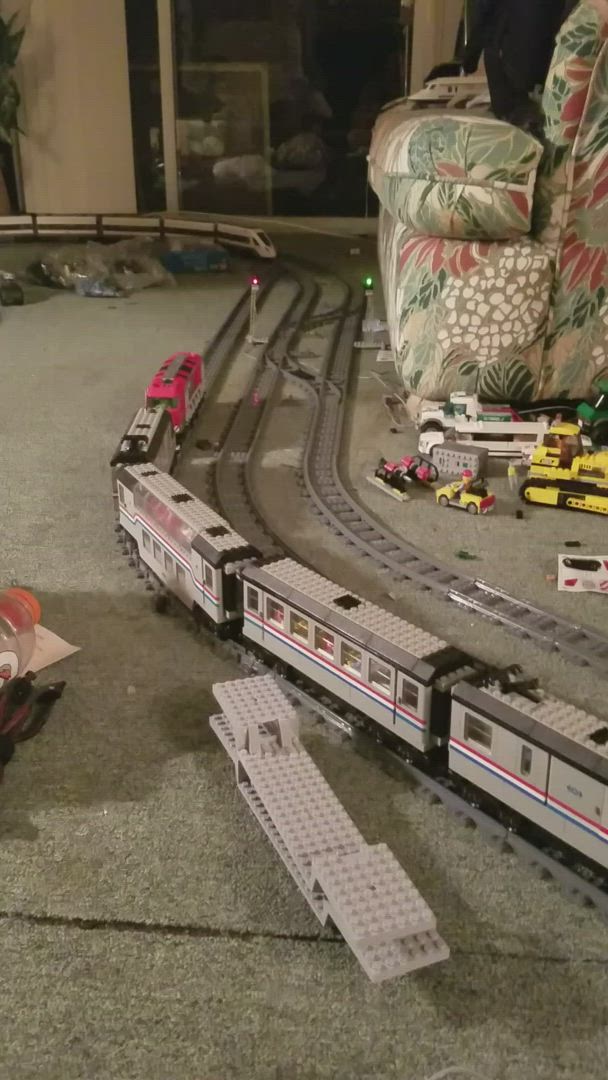This indoor photograph captures a detailed scene in a living room characterized by light gray short pile carpet flooring. Dominating the frame is an extensive toy train setup consisting of three parallel gray tracks arranged in an S-like pattern. A noteworthy feature of the image is the intricate Lego train set on these tracks. The Lego train cars are light gray adorned with red, white, and blue horizontal stripes, with some displaying black windows and Lego tops. Highlighted are a red engine car and a distinctive red and silver caboose among other passenger cars with multiple windows.

On the upper right side of the room, a fabric couch with abstract floral designs in greens and reds sits against the backdrop, partially cluttered with additional train pieces. These scattered train components include yellow construction trucks, more train track segments, and other vehicles that seem to be part of the Lego set. Notably, a spilled Gatorade bottle with a white "G" symbol and an orange cap lies on the carpet nearby, adding to the casual and lived-in ambiance.

Further enhancing the scene's homely feel, a glass door reflects the room's interior, and more toy vehicles can be seen spread around, adding to the overall sense of a playful, child-centric space.